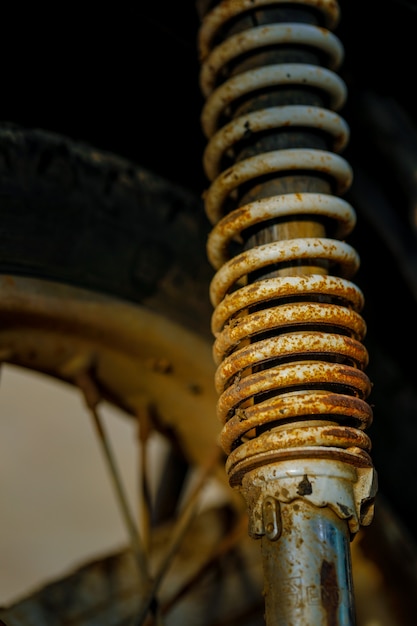The image depicts the undercarriage of a vehicle, focusing primarily on a heavily rusted suspension shock absorber. The shock consists of a silver pole, with a once-white metal spring spiraling around it from about a quarter of the way up to the top, now significantly corroded, with the white paint deteriorating to reveal orange rust. The spring appears tighter at the bottom and looser towards the top. In the background, there is a thick, potentially motorcycle or vehicle tire, characterized by its black rubber exterior and a rusted metallic frame featuring spokes; one of the spokes appears to be unattached. The setting seems dark, possibly inside a dimly lit building or museum, making it challenging to discern other details. A beige piece of fabric lies on the ground near the wheel, adding to the sense of neglect and disrepair in the scene.